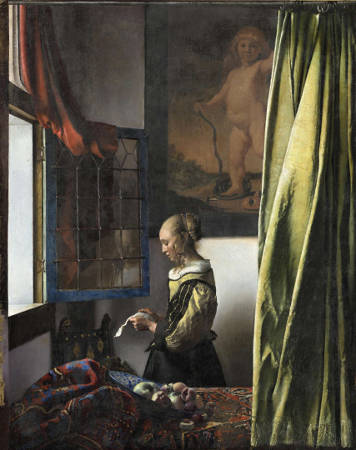This is a detailed painting depicting a woman in a classical 1800s-style dress, featuring a green top and black skirt, standing in a well-lit bedroom. She is positioned next to a bed adorned with a colorful mishmash of red, blue, and green blankets. The room is warmly illuminated by the sunlight streaming through an open window with a blue frame and small square panes, situated to the left of the scene. A red curtain, draped from the upper left corner, adds a touch of vibrancy beside the window. Opposite, on the right side of the painting, a long green curtain hangs, reaching from the ceiling to the floor. 

The woman, her blonde hair neatly styled in an elegant bun, holds a letter in her hands and gazes downwards at it with a somber expression. The backdrop behind her includes a conspicuous, large painting of a naked child, possibly an angelic figure or a baby, with distinctive hair and one hand extended towards the sky while the other holds a stick. This artwork adds a layer of peculiarity and intrigue to the composition, further enriching the scene with its historical and emotional depth.